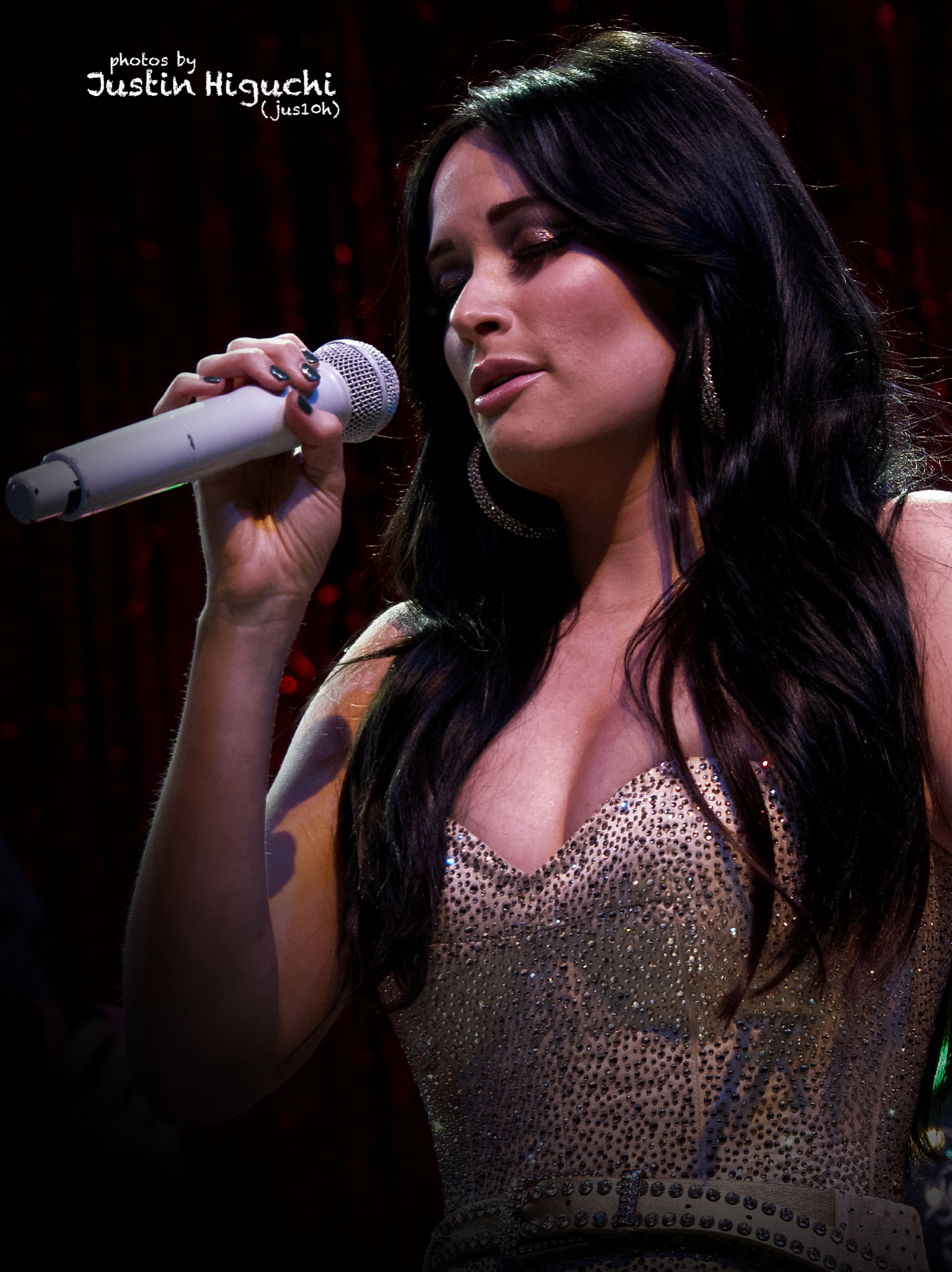The photograph depicts a close-up of a woman passionately singing into a light gray microphone with closed eyes, suggesting she is deeply immersed in her performance. The singer, possibly Kacey Musgraves given her long, wavy dark brown hair and stunning looks, exudes beauty and confidence. She is adorned in a low-cut, golden, sparkly bodice embellished with metal studs, paired with what appears to be a glittery white belt. Her dark hair cascades down to her chest, framing her face which is enhanced with heavy makeup and lipstick. Her painted nails, a dark blue-black color, add a touch of edginess to her look. The background is primarily black, featuring subtle hints of red and a small green splotch near the bottom right. The top left of the image bears a watermark reading, "Photos by Justin H-I-G-U-C-H-I."